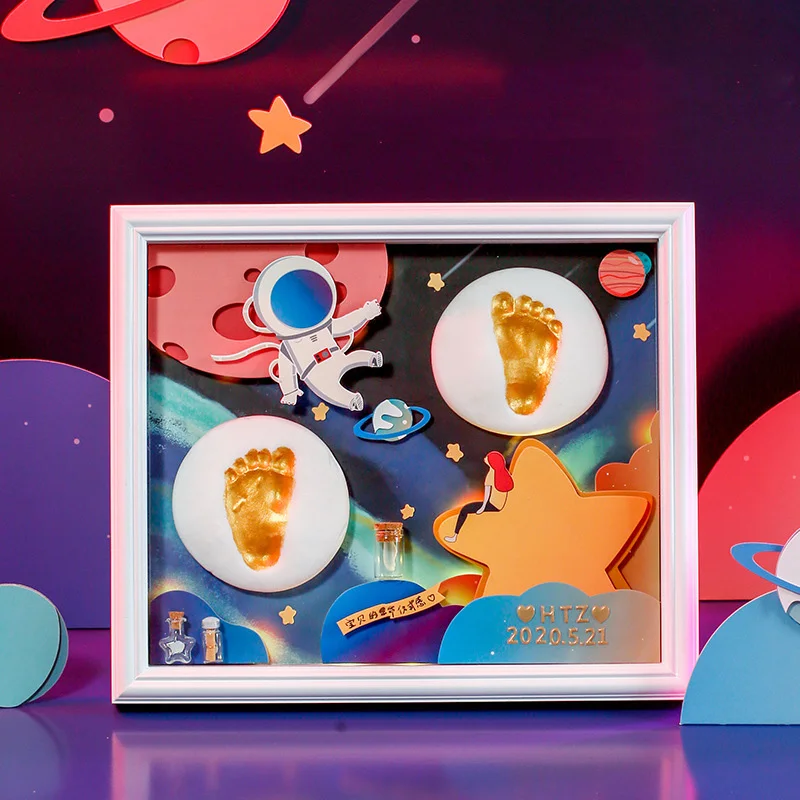In this detailed and whimsical image, we have a space-themed keepsake centered around the golden footprints of a baby. The footprints are elegantly imprinted on two white circles, marking a significant date: May 21, 2020, alongside the initials "HTZ". The scene is set against a vibrant, starry background, featuring a plethora of colorful elements. A girl with flowing red hair sits on the edge of an orange star, gazing dreamily. Nearby, a cheerful childlike astronaut, dressed in white and blue, seems to float toward the Earth, which is encircled by a glowing halo. The backdrop is decorated with cosmic details like Saturn, shooting stars, and multiple planets in hues of blue, pink, and red. Overhead, Saturn makes another appearance, while the pink Jupiter peeks from the side. Tiny, somewhat indistinguishable images in one corner suggest elements like a baby bottle. This imaginative tableau is set against a wall painted to match the celestial theme, featuring stars, planets, and even some Chinese characters, providing a nostalgic yet playful memorial of the child’s birth.